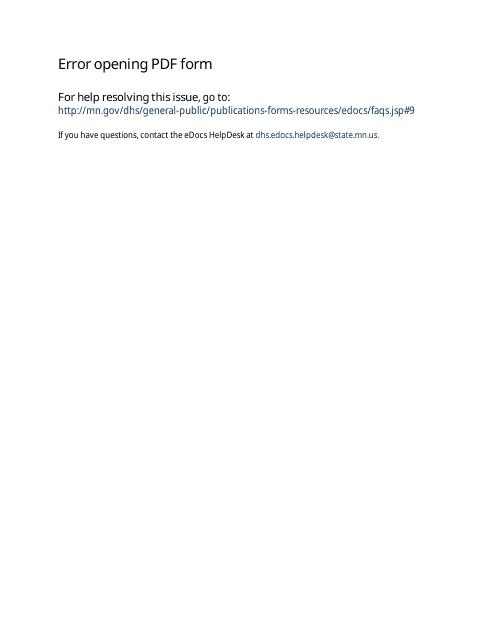"Error: Opening PDF Form

Approximately two inches below the title, there is a message that reads: 'For help resolving this issue, go to the following link: http://mn.gov/DHS/general-public/publications/forms-resources/eDocs/faqs.jsp#9'. The link is colored blue, indicating that it is clickable.

If you have any questions, you are advised to contact the eDocs helpdesk via email at dhs.edocs.helpdesk@state.mn.us."